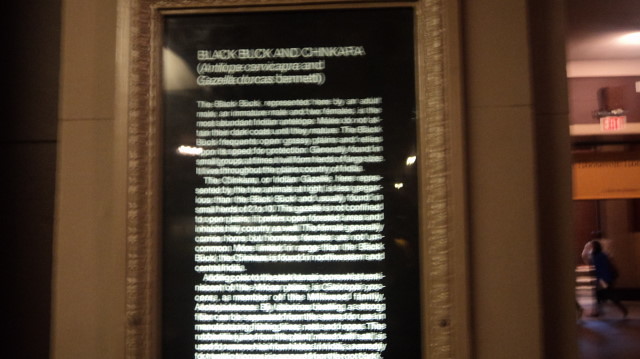In this image, a prominent black sign with white text is centrally displayed, listing the words "black," "buck," and "chinkara." The finer details under these words are unclear. The sign is elegantly framed in brown wood that harmonizes with the matching wall. On the right side, there are double doors with an illuminated exit sign above them. Below the sign, a figure wearing a blue shirt appears to be either running or walking towards the left. Additionally, from the upper right corner of the image, a light source casts illumination across the scene. Above the exit sign, there is a speaker.